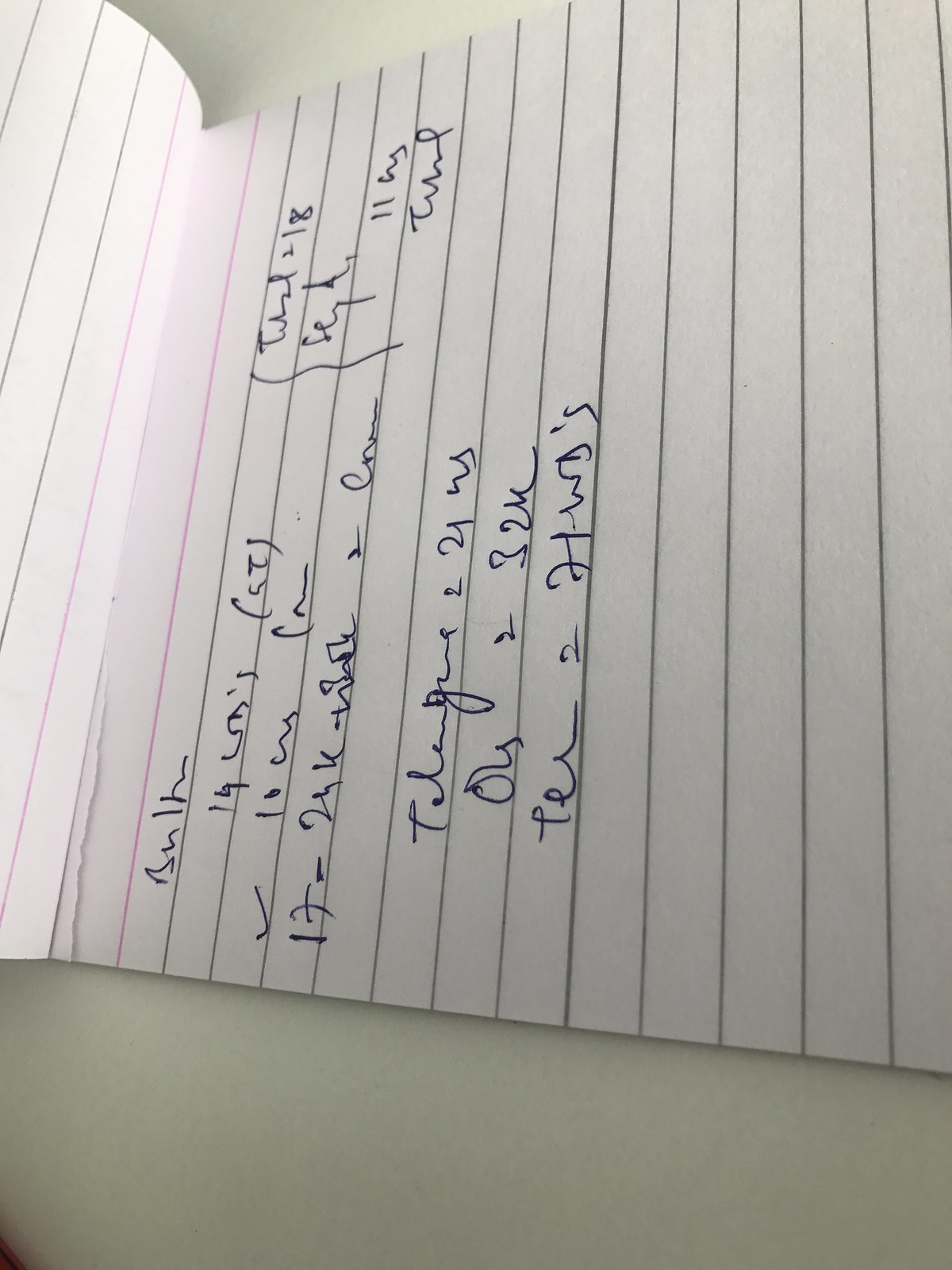This image features a sheet of white notepad paper with a ripped edge, indicating it was torn from a notepad. The paper includes eight lines of handwritten text, which appears to be an attempt at solving a mathematical problem. The handwriting is somewhat difficult to read, and while the symbols and terminology used in the calculation are obscure to the viewer, it is clear that it involves mathematical equations. At the top of the page, there is a term that looks like "bulk," though this is uncertain. The notepad is college-ruled, and there is space at the top for a title, further confirming that it is a sheet from a notepad and not an index card.